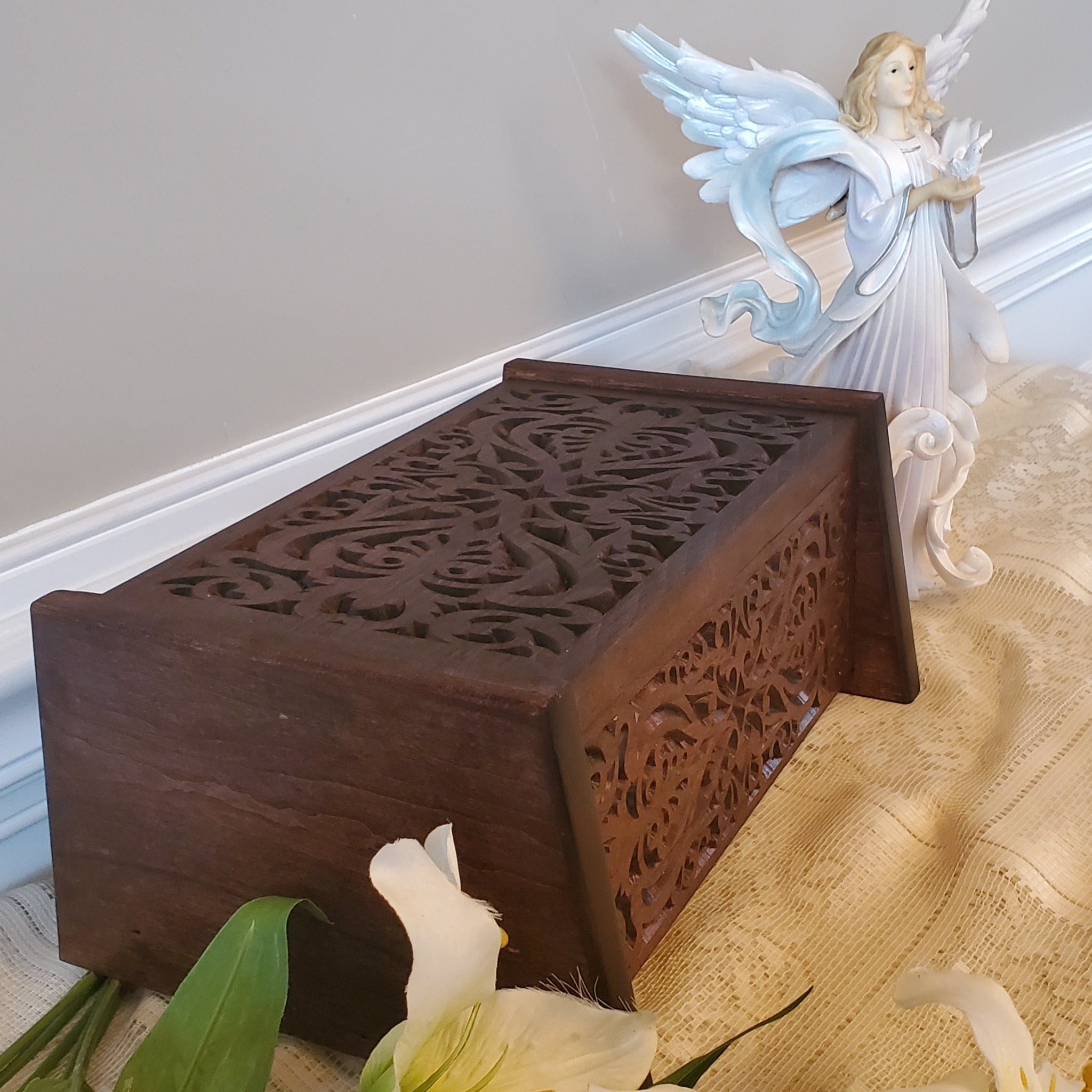The image depicts a scene composed on a table adorned with an ochre-colored lace tablecloth. Dominating the center of the table is an intricately carved dark wooden box, which might be a decorative or ceremonial urn. The carvings feature an ornate pattern, possibly leaves, demanding high craftsmanship. To the right of this box stands a porcelain angel figurine. The angel is depicted with white flowing wings and gown, a light complexion, and blonde hair, cradling a small ceramic dove in its cupped hands. On the left side of the box, a delicate orchid emerges, showcasing its vibrant green leaves and a striking white bloom. The background is marked by a gray wall and white railing, providing a neutral, yet elegant setting for the objects displayed.